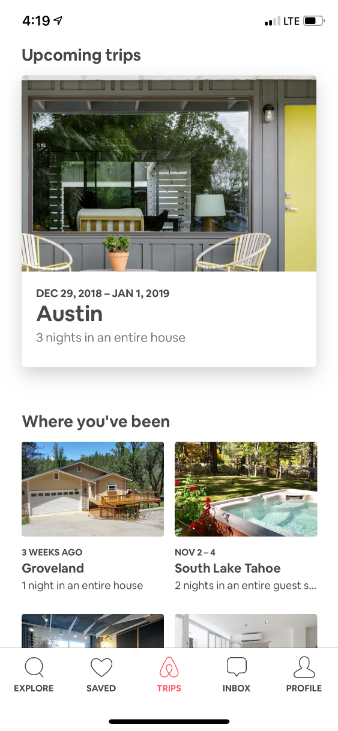### Detailed Caption:

The screenshot captures a page from a home screen related to travel plans, set against a stark white background on the top left corner. The time displayed is 4:19, accompanied by a small arrow pointing upwards and to the right. To the right side, a battery icon indicates it's about 70% full, with the top portion in black and the bottom in white. Adjacent to the battery icon, "LTE" is displayed, followed by a Wi-Fi signal icon showing two black bars and two gray bars.

Beneath the time, the text "Upcoming Trips" is prominently featured. Below this header, there’s a detailed image of a house. The house's exterior includes a gray wall spanning the top, the left side, and across the bottom. About an inch from the right side, the wall extends upwards and curves over at the top. 

In the center of the gray wall, a large window is visible. In front of this window, a chair is placed in both the left and right corners, flanking a potted plant with a small green bush. A yellow door is situated on the right side of the house, just below a light fixture positioned slightly to the left of the door. Underneath these elements, bold text displays the location as "Austin," along with smaller, black text indicating the duration of the stay in nights.

Additionally, there’s a segment labeled "Where You've Been." It features a picture of another house with a tan exterior, a garage, and a driveway, surrounded by trees and a sky backdrop. Further details include the length of the previous stay, location, and number of nights.

In the bottom right of the page, there's an image of a jacuzzi that spans about halfway up the screen, with a green lawn above it. Below this point, the details of the stay, location, and duration are outlined.

Finally, there’s a navigation menu at the bottom of the screen, displaying five icons in a row. From left to right, these icons include:
1. A compass-like "Explore" icon.
2. A heart labeled "Saved."
3. A red Airbnb logo labeled "Trips."
4. A text message box icon labeled "Inbox."
5. A user profile icon marked "Profile."